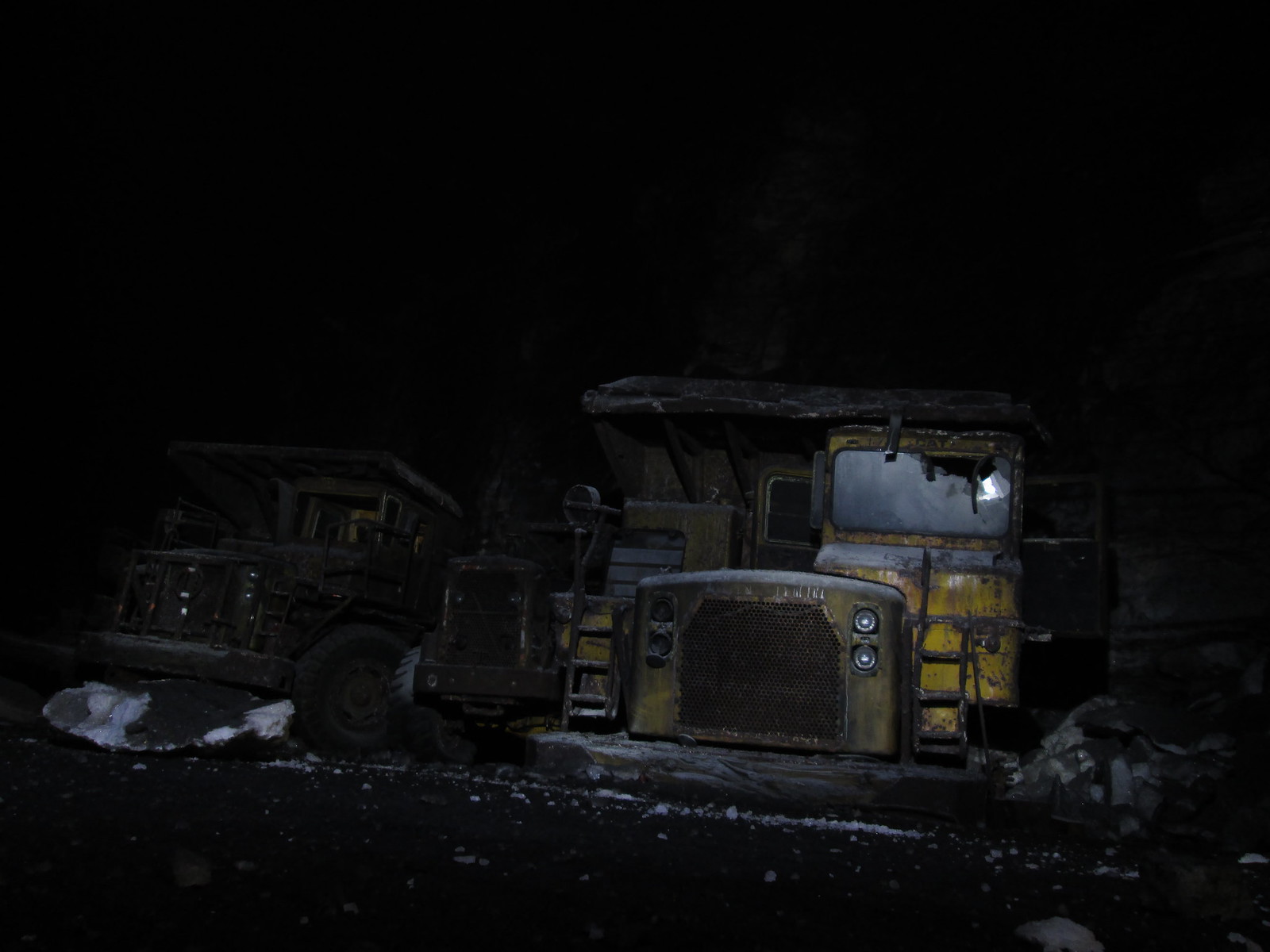In this nighttime photograph, illuminated by a streetlight or parking light, we see a collection of old, distressed work vehicles parked closely together, possibly in a lot or an abandoned site. The scene is quite dark, with a dim, ambient glow revealing more detail on the vehicles. On the left side, a large, rusted dump truck is visible, its original yellow paint barely discernible amid the layers of rust and dirt covering it. This truck is muddied and caked in grime, and features a busted windshield along with its four headlights and characteristic grill. To the right, there is a smaller, equally dilapidated vehicle resembling a small tractor, lacking a roof or cab, and appearing more diminutive in size. Amidst these two, there's another severely rusted structure which might be a third vehicle or possibly some sort of machinery, adding to the scene's overall decrepitude. The vehicles are set against a dark background that makes it challenging to distinguish additional elements, contributing to the eerie, forsaken feel of the photograph.